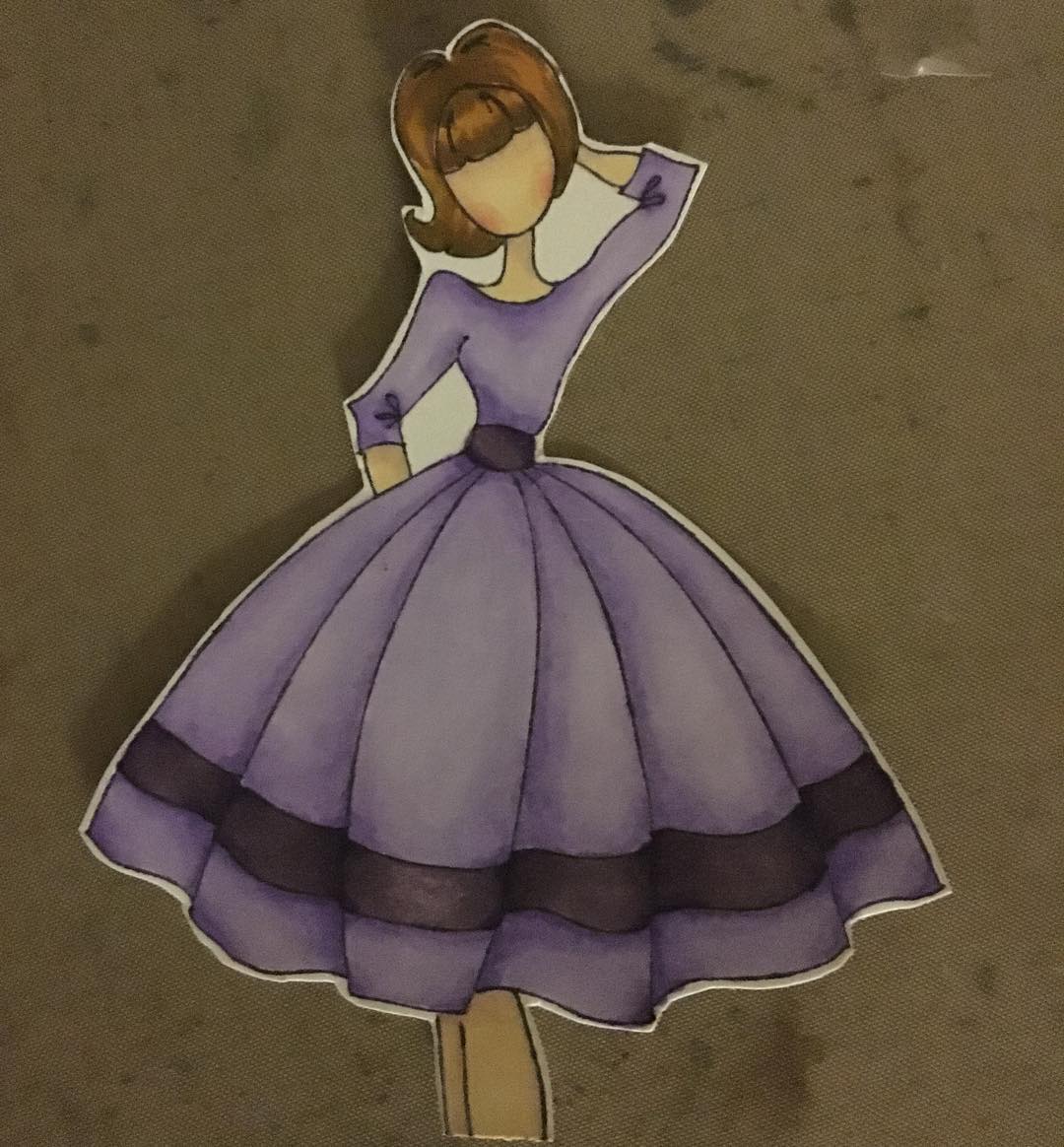This is an image of a paper doll or cutout of a woman dressed in a 1950s-style outfit, positioned on a surface that appears to be a dark, marble-like background with brown and green mottled markings. The cutout features a woman with no facial features, dressed in a light purple-violet dress with a darker purple band at the waist and near the knee-length hem. The flowing, full-pleated dress is complemented by a 50s-inspired hairstyle, which is tall on top, falls to the sides, and has front bangs. The woman is posed with one hand behind her head and the other arm behind her back, giving her a playful, stylized appearance. The entire scene has a watercolor feel, adding to the artistic and vintage charm of the image.